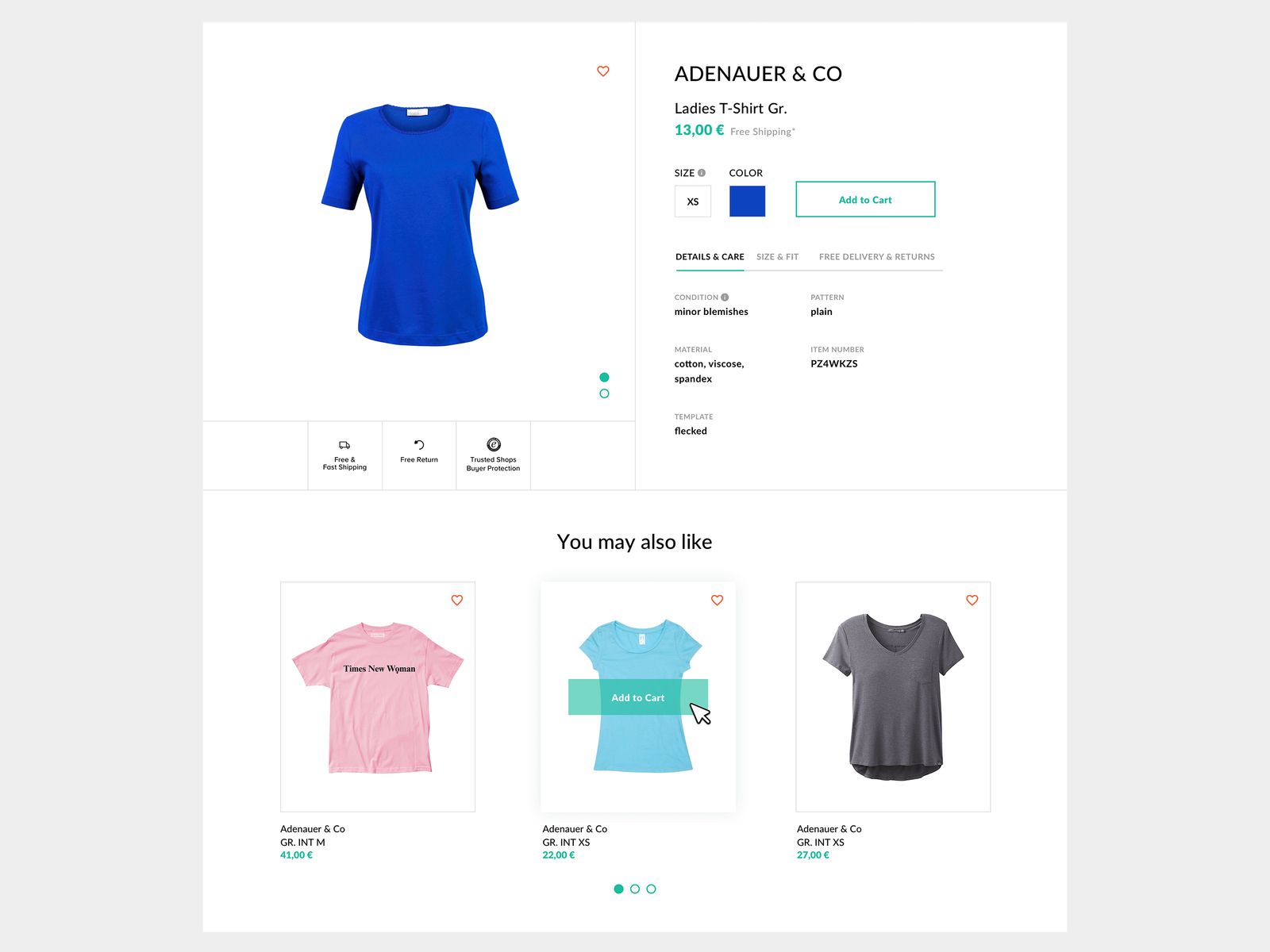This image appears to be a snapshot of a clothing website, specifically showcasing a women's t-shirt. At the top center-right of the image, the brand name "Aidenarer & Co" is displayed in bold black text. Directly beneath the brand name, the product title "Ladies T-Shirt GR" is noted in smaller text. The price, listed in British Pounds, is £13.00 and is accompanied by a "Free Shipping" label. 

To the left of these text elements, a large square displays the actual product—a bright blue t-shirt. Adjacent to the product image, on the right side, options for selecting size and color are visible, along with an "Add to Cart" button prominently featured in a green rectangular box.

Below the product options, there are several category tabs labeled "Details and Care," "Size and Fit," and "Free Delivery and Returns," separated by a horizontal line. 

Towards the bottom middle of the image, three additional product options are showcased in small square frames. The product on the bottom left is a pink shirt, the middle product is a light blue blouse, and the right product is a light gray blouse—all designed for women.